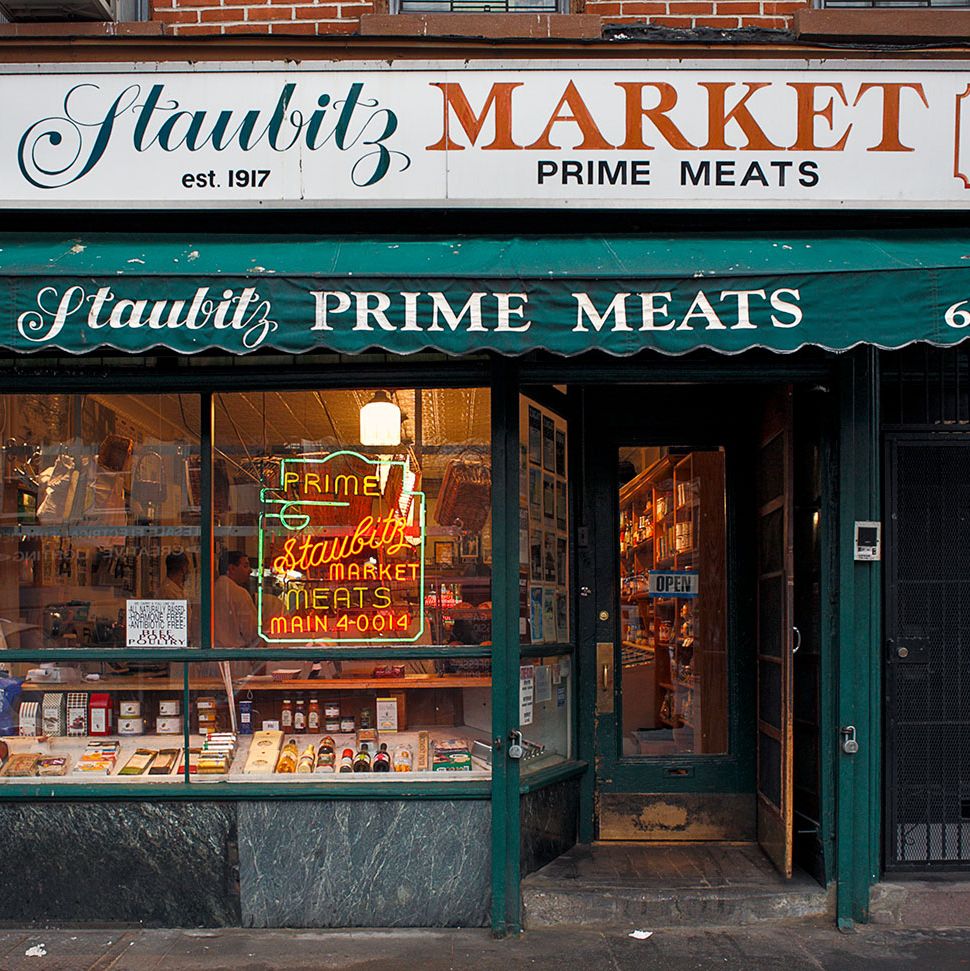The image depicts the entrance of a butcher shop named "Stout Butts Prime Meats," which is housed in a red brick building. The storefront features a green awning with white text stating "Stout Butts Prime Meats." Above the awning, a white banner with black text reads "Stout Butts Market," with "Established 1917" and "Prime Meats" underneath. The open doorway reveals a wooden-framed screen door with chipping green paint, a brass handle, and a sign stating "Open" in black text. Next to the doorway, on the left side, a neon sign illuminates with green and yellow text: "Prime Stout Butts Market Meats Main 4-0014."

The shopfront also displays a variety of products, including bottles and other containers. Inside the store, you can see two employees dressed in white butcher gowns working behind a wooden counter. The interior showcases wicker baskets, wooden shelves, and produce, while the exterior includes a gray, slightly dirty concrete sidewalk and steps leading up to the entrance.